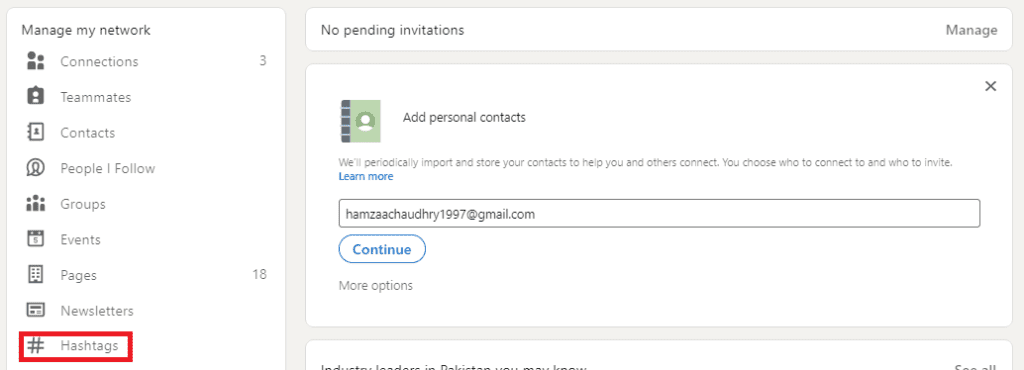In this detailed screen capture of a computer page, we observe what seems to be an organization software interface. On the left side of the screen, there is a navigation panel written in black and white titled "Manage my network." This panel contains several links organized sequentially from top to bottom: Connections, Teammates, Contacts, People I Follow, Groups, Events, Pages, Newsletters, and Hashtags.

Moving towards the right, another small window appears, also in black and white, with the message "No pending invitations" followed by the option to "Manage." Below this section, there is a window titled "Add personal contacts" stating, "We'll periodically import and store your contacts to help you and others connect. You choose who to connect to and who to invite." This panel includes a clickable "Learn more" link.

At the bottom of this window, a Gmail address is visible: "HamzaChaudhry1997@gmail.com," accompanied by a link labeled "Continue" which likely serves to proceed with the import or connection process. The design and layout seem structured to help users efficiently manage and grow their network by providing various tools and options.